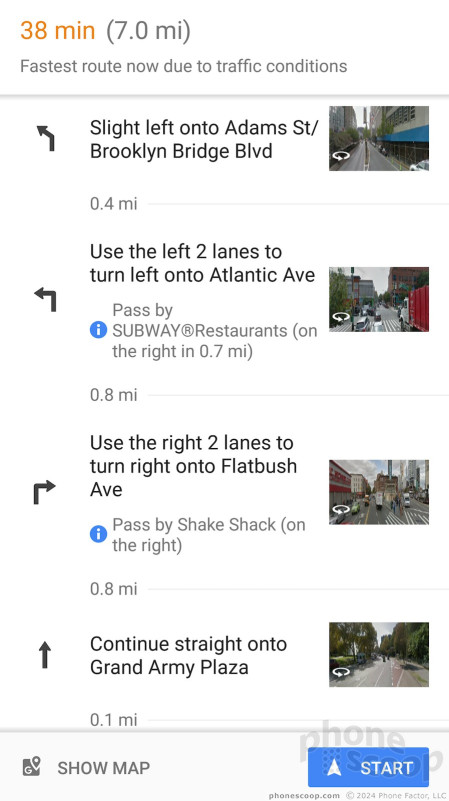The caption given by voice has been cleaned up and restructured for clarity and detail:

---

Travel Time and Directions from Adams Street, Brooklyn to Grand Army Plaza

Due to current traffic conditions, the fastest route to cover 7 miles is estimated to take 38 minutes.

1. Slight left onto Adams Street/Brooklyn Bridge Boulevard.
    - Continue for 0.4 miles.
    - (An image of the street with a black arrow indicating the direction is shown here).

2. Use the left two lanes to turn left onto Atlantic Avenue.
    - Pass by Subway restaurants on the right after 0.7 miles.

3. Use the right two lanes to turn right onto Flatbush Avenue.
    - Pass by Shake Shack on the right after 0.8 miles.
    - (An image of Flatbush Avenue is shown here).

4. Continue straight onto Grand Army Plaza.
    - Proceed for 0.1 miles to reach your destination.
    - (An image of Grand Army Plaza is shown here).

Interesting Note:
Where I live, in 38 minutes you could probably travel around 20 miles or even 38 miles in 38 minutes, which is significantly quicker.

At the bottom of the directions, there's an option to "Show Map" and a "Start" button for navigation.

---